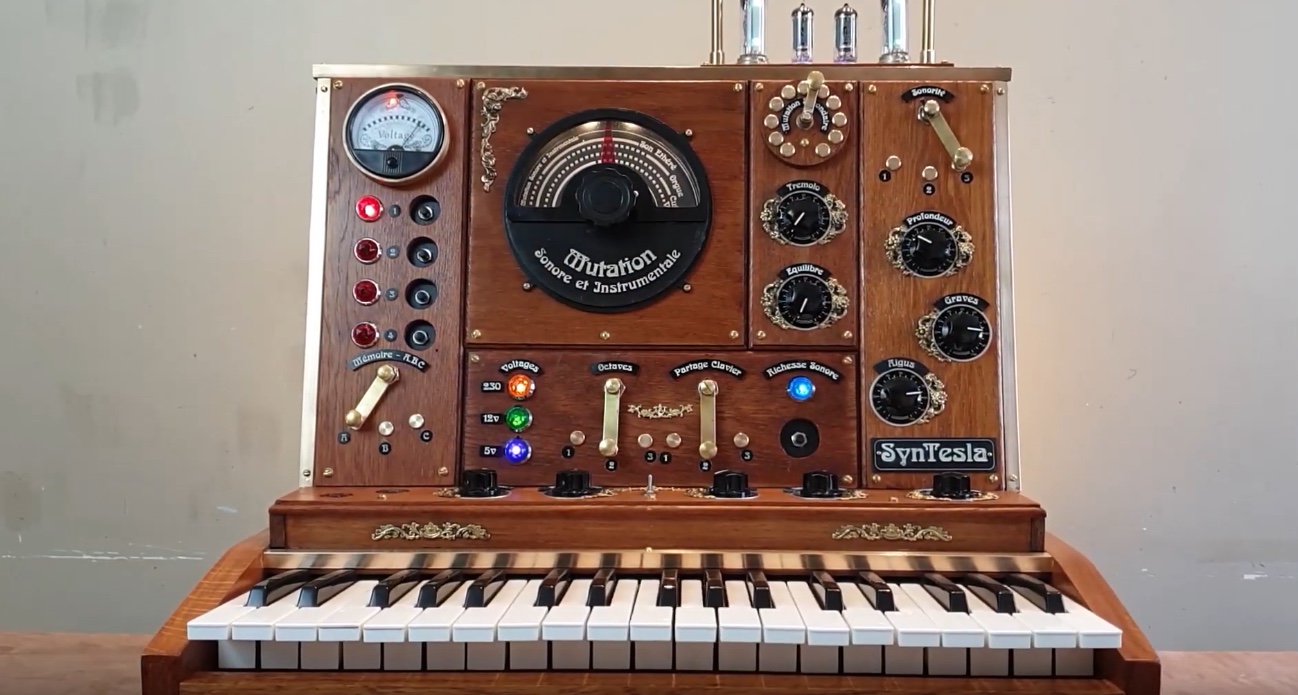The image depicts a vintage-looking musical instrument resembling an organ keyboard, housed in a medium honey-colored wooden case. The keyboard section features white and black keys, with approximately 15 black keys visible. Above the keyboard, numerous gauges, dials, and colored buttons are present, including orange, green, purple, red, and blue lights. A prominent black dial labeled "Mutation Sonore Instrumento" sits centrally amidst these controls. Additionally, the apparatus has decorative carvings and some pipes extending from the top right-hand side. The name "Syntesla" is inscribed on the bottom right of the instrument, hinting at its brand or model. The background consists of a plain gray wall, accentuating the intricate details and vintage charm of the equipment.